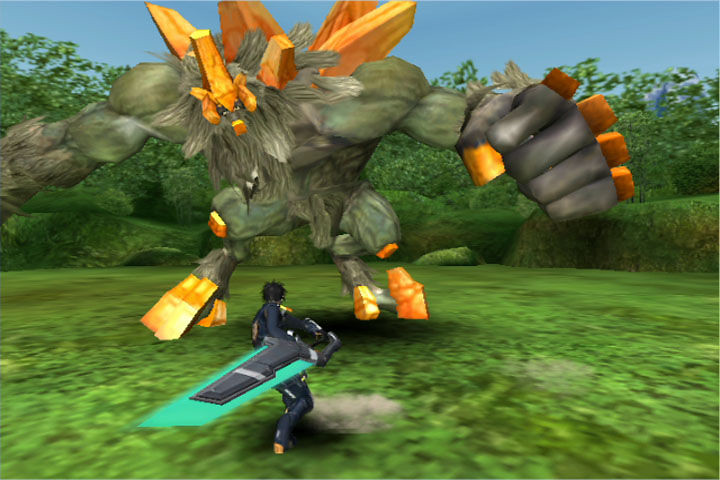This vivid color photograph resembles an AI-generated image or a screenshot from a video game. It features a dynamic scene set against a backdrop of a clear blue sky with lush green trees and shrubs below. In the foreground, a varied shade of green grass spans the bottom of the image, setting the stage for the characters present. Central to the scene is a person seen from behind, clad in a long black suit and sporting black hair. This individual holds a green and blue surfboard under their right arm. Dominating the scene in front of them is a towering, monstrous figure. This creature boasts large gray limbs composed of massive circular segments, embellished with striking orange crystal-like protrusions on its head, back, fists, and legs. The creature's formidable appearance is emphasized by its exaggerated muscle tone and distinctive orange features, which add a surreal, game-like quality to the overall image.